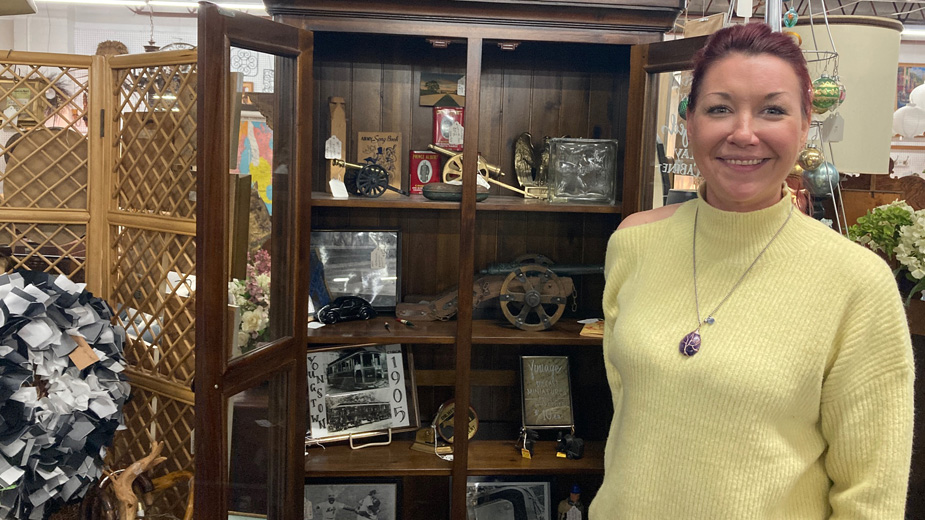A woman stands proudly in front of an antique wooden curio cabinet with opened glass doors, revealing a collection of miniature cannons and black and white photographs. One prominent photograph reads "Youngstown, 1905" and depicts a historical scene. The woman, smiling warmly, wears a soft yellow sweater and a necklace with a gem pendant. Her hair is pulled back, and she exudes a sense of pride, possibly showing off the curated items. To her left is a decorative wooden screen, and behind her, decorative elements like flowers or wreaths and a lampshade further enrich the vintage ambiance. This indoor setting, likely in an antique shop or at a flea market, encapsulates a fondness for historical memorabilia.